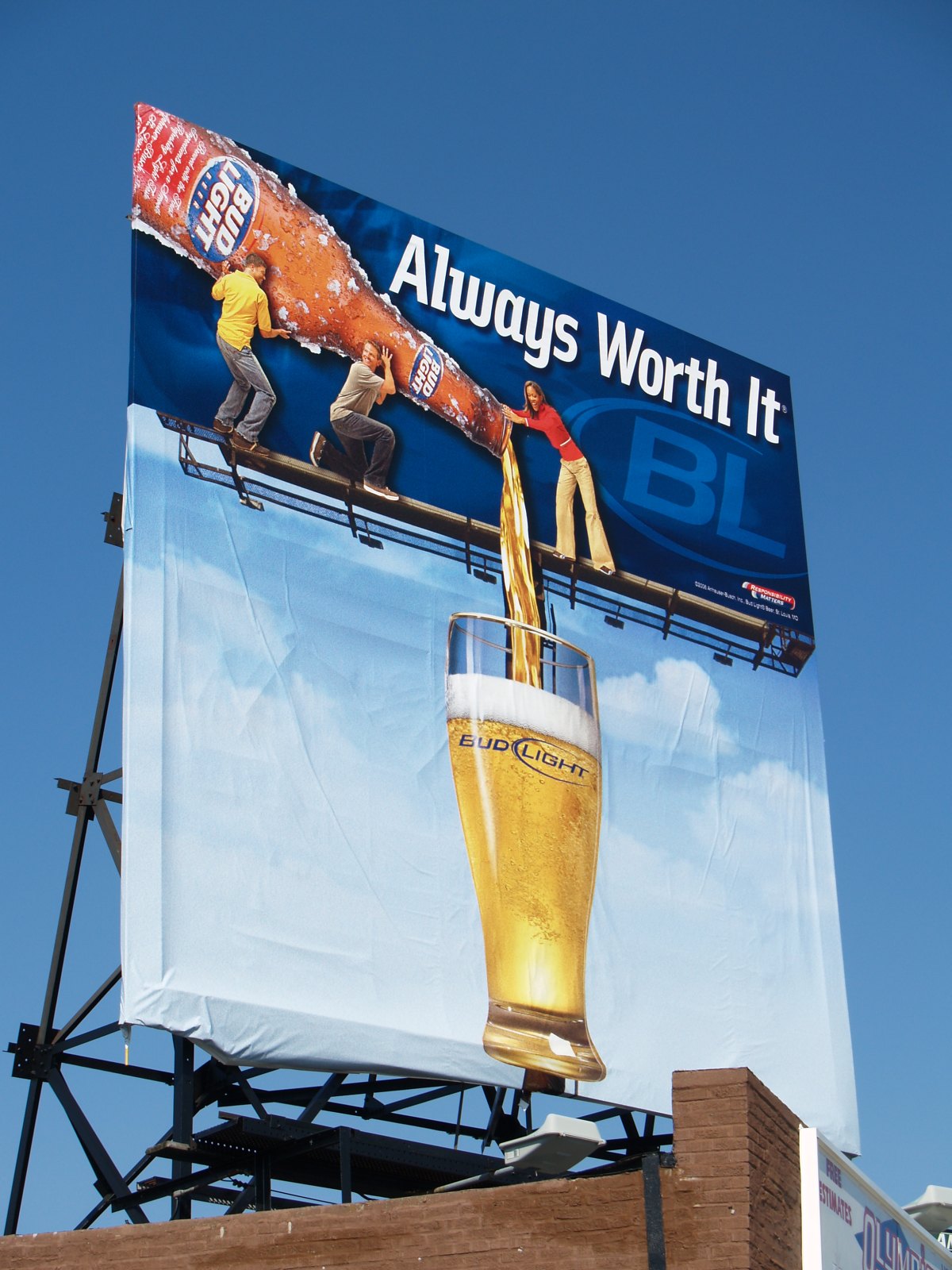The billboard for Bud Light is captivating against the stunning, cloudless sky that transitions from a dark to medium blue. Rectangular and tilted slightly upwards, the billboard draws your attention with its dynamic imagery and vibrant colors. 

In the upper left corner, there is a frosty brown Bud Light bottle, adorned with significant amounts of ice. The bottle appears quite appealing, almost 'cute,' as it glistens with the frozen condensation. Two men are in the scene; one is kneeling on one knee in the foreground, while the other stands behind him, sporting jeans and a yellow t-shirt, holding up the frosty bottle with both hands in a celebratory manner.

Below the bottle's mouth stands a lady, guiding the golden liquid into a clear glass that prominently displays the Bud Light logo. The liquid pours smoothly, crowned with a foamy white top, and contrasts beautifully against the white background of that section of the billboard. The backdrop appears to be made of a slightly wrinkled fabric or canvas, adding texture and depth to the advertisement.

Situated atop a medium brown brick building, the billboard seamlessly integrates with its urban surroundings while standing out vividly against the picturesque sky. It's not just an advertisement but a visual spectacle that commands attention and admiration.